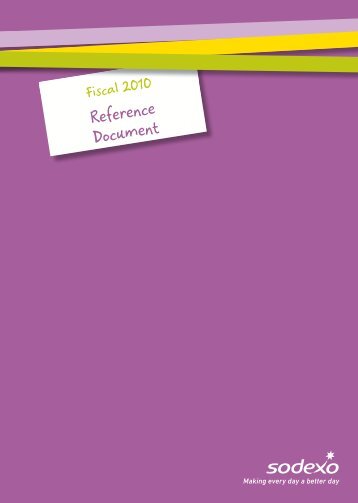The image depicts a lavender-colored poster board, commonly used for tacking notes. The board features three ribbon-like stripes at the top: one in light lavender, one in deep yellow, and another in medium green, arranged diagonally and slightly off-center. Tucked under these ribbons is a white tag that reads "Fiscal 2010" in green script and "Reference Document" in lavender script. At the bottom right corner, the brand name "Sodexo" appears, accompanied by its slogan "Making Every Day a Better Day." The Sodexo logo includes a distinctive white star at the right point of the 'X'. This poster board likely serves as an organizational tool, possibly used during meetings to display important financial documents for the year 2010.